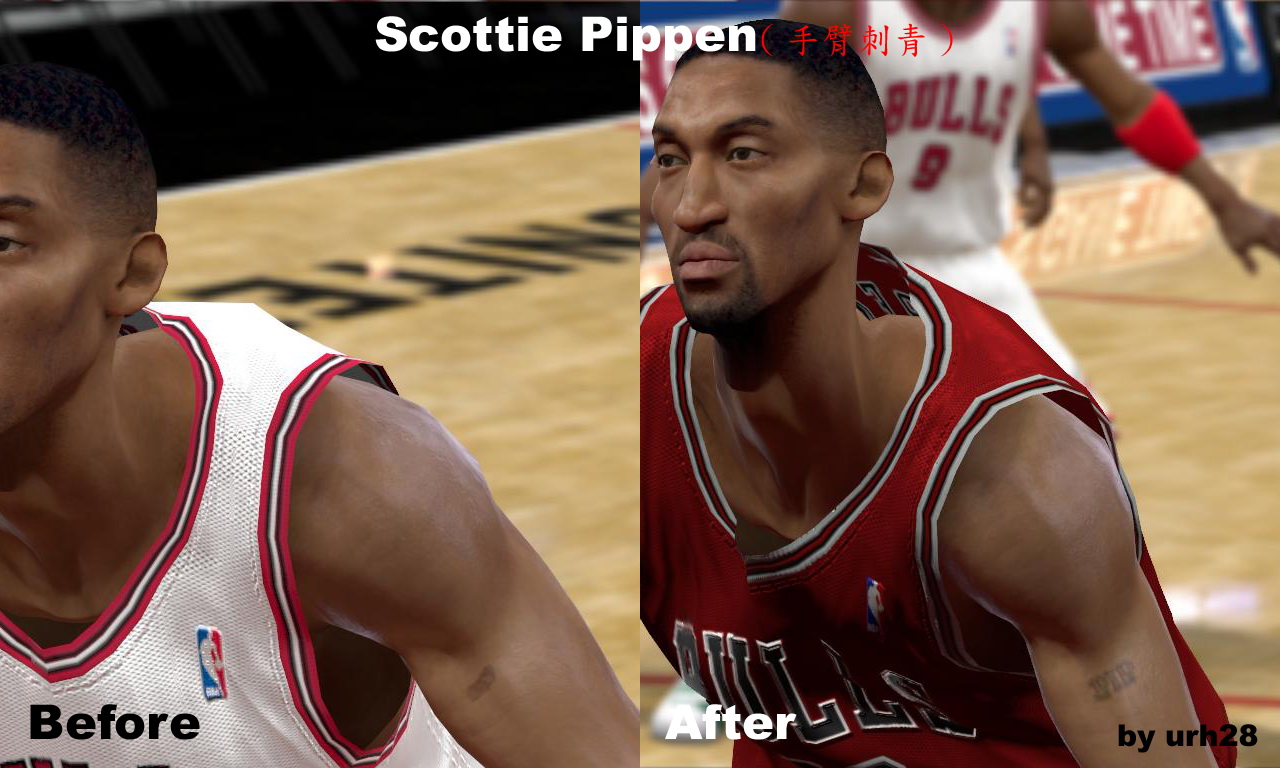The image consists of two side-by-side screenshots from a video game, both featuring the basketball player Scottie Pippen under the text "SCOTTY PIPPIN" in white at the top center. The left image, labeled "BEFORE" in black text at the bottom left, shows Pippen running to the left, wearing a white basketball jersey adorned with red, white, and black stripes on the hem, neckline, and armholes. The background features hints of a basketball court and additional colors including light brown and blue. 

In the right image, marked "AFTER" in white text at the bottom left, Pippen is seen wearing a red jersey with the word "BULLS" prominently on the front. His left shoulder slightly overlaps with the torso of another player wearing a white jersey with the number 9 and the "BULLS" logo. The court is visible to the right of Pippen in this image. Notably, the bottom right of this photograph contains the text "BUY URH 2 8." This combined presentation appears to compare before and after states of the player within the video game's stylized setting.